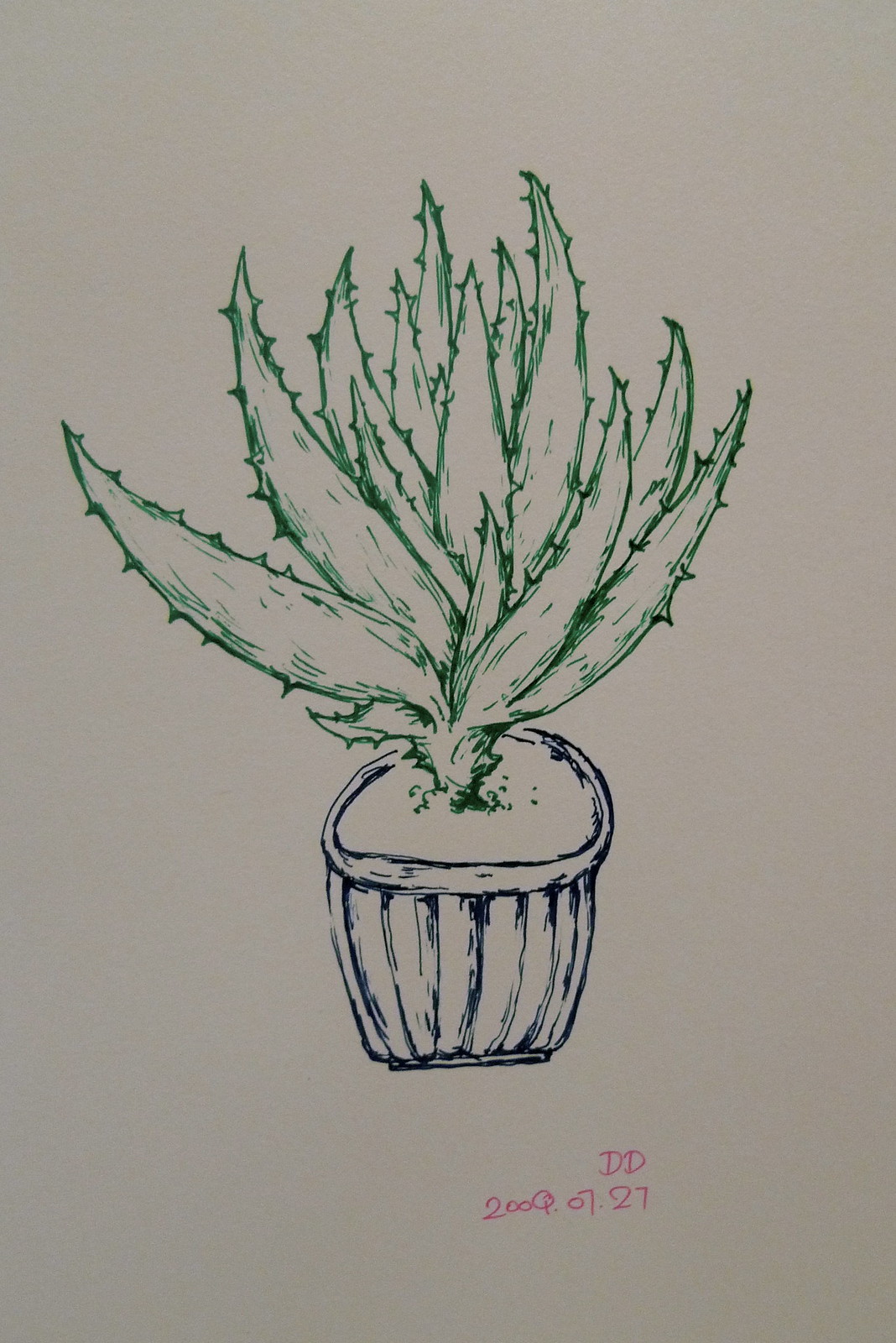A meticulously detailed sketch of a plant is presented against a gray paper background. At the base of the sketch, the notation "DD" appears in a subtle pink hue alongside the sequence "200Q" and the number "0727." The lower portion features a vase-like shape, outlined in bold black, with a distinctive ring encircling its top. From this vase, approximately 12 to 15 elongated green leaves emerge, each intricately outlined and springing upward with vivid dynamism. The overall minimalist aesthetic is enhanced by the consistent gray backdrop, which serves to highlight the intricate details and subtle color contrasts within the sketch.